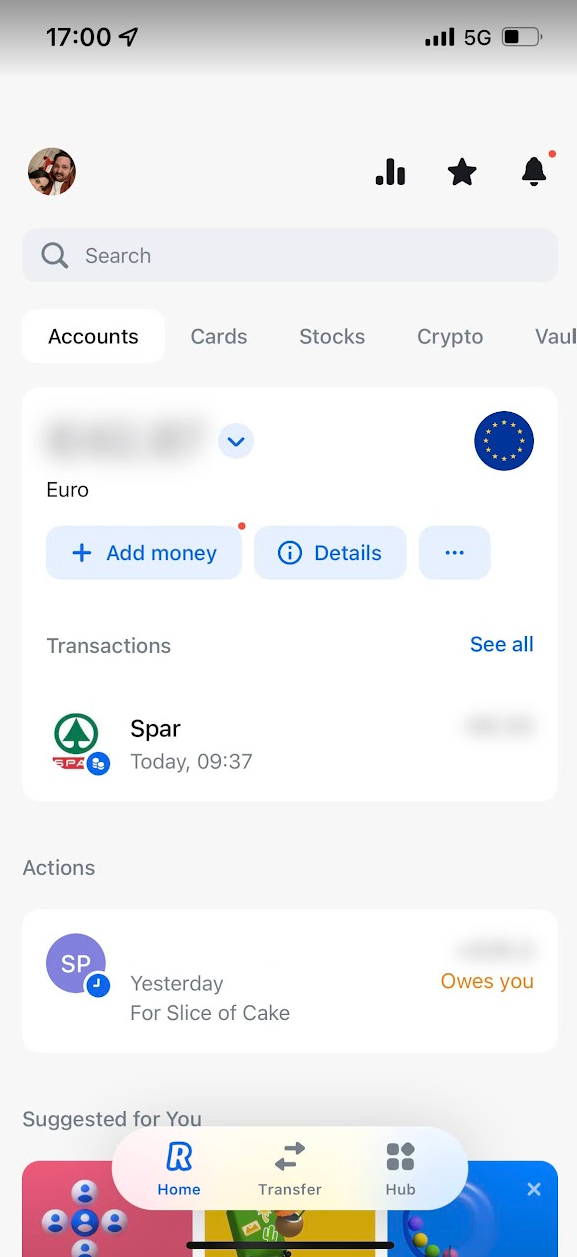This is a detailed screenshot of a finance application interface. In the top left corner, there is a profile picture indicating that the user is logged in. Adjacent to the profile picture, there are a series of unidentified icons, one of which appears to be for notifications. Directly below these icons is a search bar devoid of any search terms.

Following the search bar, a main menu is displayed with options labeled as "Accounts," "Cards," "Stocks," "Crypto," and "Vault." The account information reveals the currency as Euros, suggesting the user is based in Europe. There are "Add Money" and "Account Details" buttons clearly visible beneath the account section.

Under this, the transactions section lists recent financial activities. The user has made a purchase at a supermarket named Spa today at 9:37 AM. A button is available to view all listed transactions.

Further down is an "Actions" section. It includes a note that the user paid for "a slice of cake" yesterday. Accompanying this note is an icon with someone's initials and the label "owes you," suggesting the app includes functionality for peer-to-peer money transfers.

Towards the bottom, there is a "Suggested for You" section with indistinct images, presumably personalized recommendations. Finally, at the very bottom of the screen, a menu bar provides quick access to "Home," "Transfer," and "Hub" options.